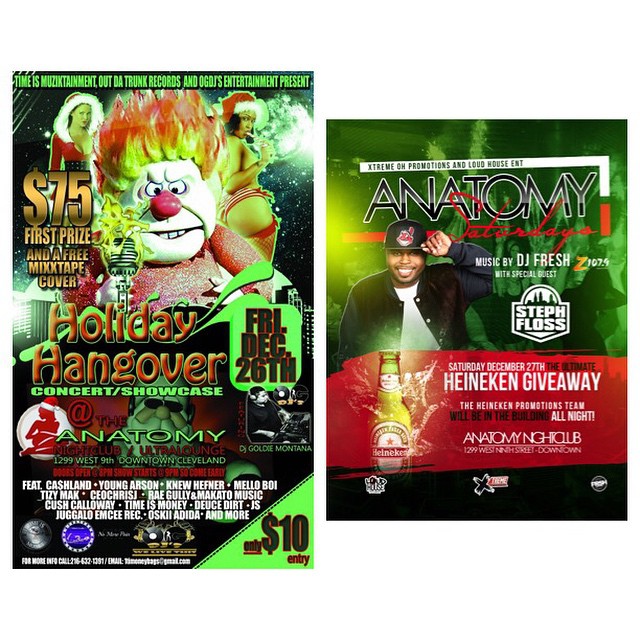This photograph features two vibrant posters advertising holiday-themed nightclub events at the Anatomy Nightclub and Ultra Lounge at 1299 West 9th Street, downtown Cleveland. 

The left-hand poster, predominantly green, presents the "Holiday Hangover Concert Showcase" scheduled for Friday, December 26th, with a $10 entry fee. At the top, it depicts a cartoonish figure resembling Heatmiser from a Santa Claus animated movie, characterized by his fiery hair, red nose, and angry expression, standing behind a flaming microphone. Surrounding him are two women clad in sexy Santa Claus outfits, one smoking a cigarette while donning a Santa hat and stockings, and the other wearing only a Santa hood. The poster highlights a $75 first prize and a free mixtape cover, and lists performers such as Cash Land, Young Arson, and New Hefner. The event is presented by Time is Musictainment Out the Trunk Records and O'Goes Entertainment.

The right-hand poster contrasts with a green background and focuses on "Anatomy Saturdays" hosted by Xtreme Old Promotions and Loud House Entertainment on Saturday, December 27th. It features a photo of Steph Floss, a black man sporting a Cleveland Indians hat, a black jacket, and a white t-shirt, presumably the special guest DJ for the night. Music is provided by DJ Fresh from Z107.9, and the event includes "The Ultimate Heineken Giveaway," indicated by the image of a Heineken bottle. The Heineken Promotions team will be present all night to enhance the festivities. The poster also includes logos for Xtreme, a company with a black globe in its logo, and Loud House.

Both posters are rich in detail and highlight special guests, performances, and engaging visuals to attract attendees to these holiday celebrations at the Anatomy Nightclub.